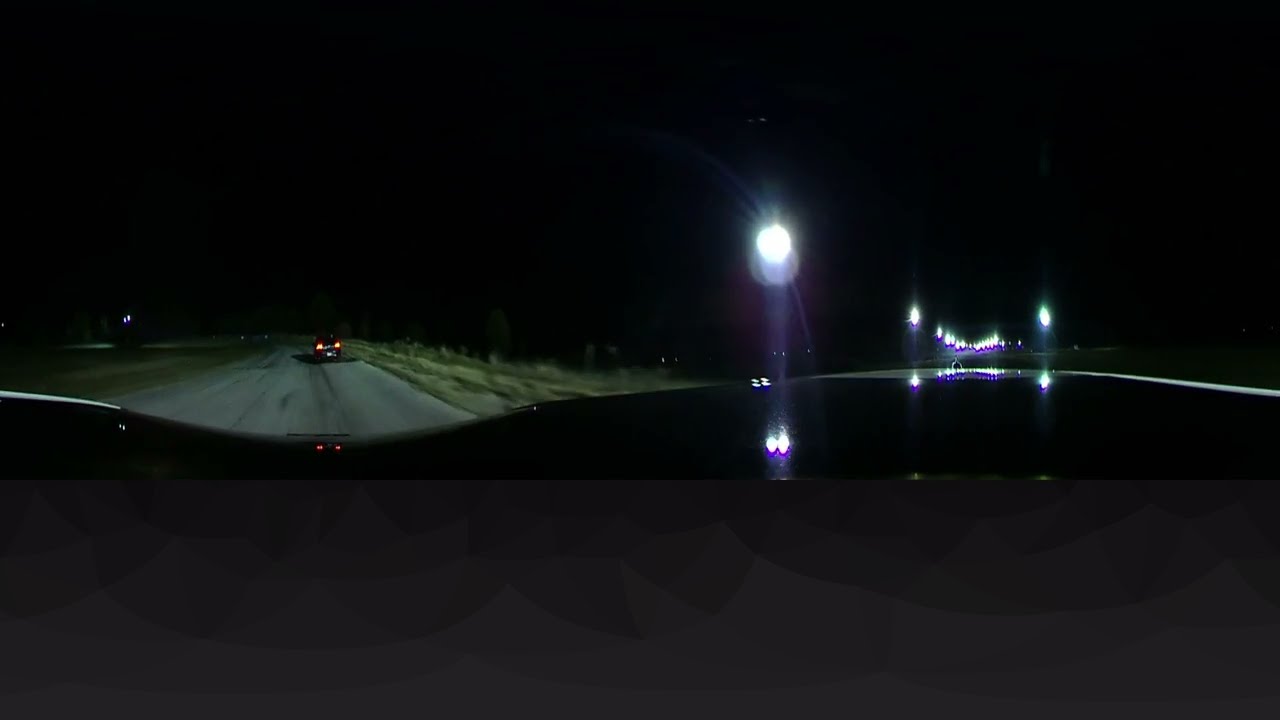In this nighttime image, the perspective is from a vehicle driving down a dark road. The photograph seems to be of low quality or perhaps distorted, possibly resembling a wraparound or 360-degree image. The central focus is the road ahead, illuminated only by the headlights of the vehicle from which the picture is taken. The sky above is pitch black without any stars, emphasizing the nighttime setting.

In front of the vehicle, there's another car with glowing red taillights, but no other vehicles, people, or animals are visible. On the right-hand side of the image, there is a line of bright yellow streetlights with a hint of purple fringing, casting light onto the dark surroundings. The pavement is a light gray color, and there is a strip of green grass along the sides of the road, adding a touch of color to the scene. The image conveys a sense of isolation and highlights the contrasting lights against the dark night.